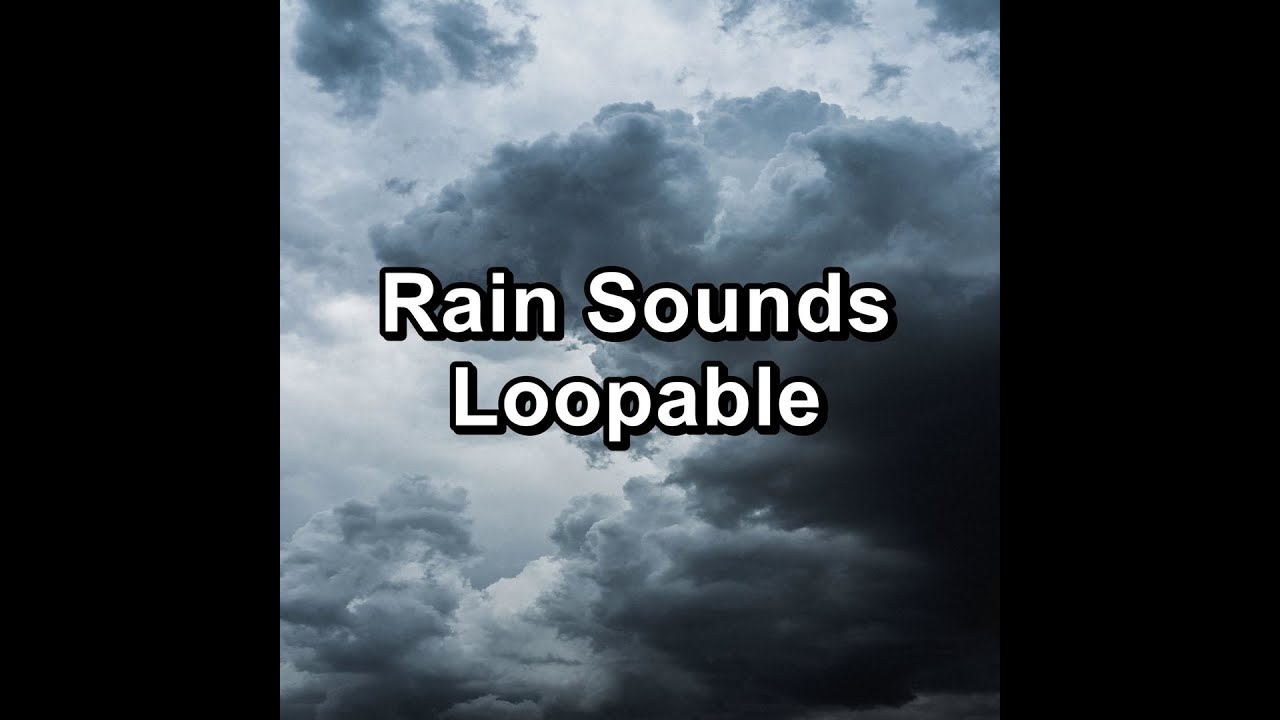In the center of this square image, bold white text with a black border reads "Rain Sounds" on the first line and "Loopable" on the second line. The background is a photograph of a cloudy sky filled with various shades of dark grey clouds. There are no visible ground elements or other objects like humans or airplanes; it's purely a sky scene. Along the left and right sides of the image, two vertical black strips frame the cloudy sky, giving the impression of boundaries within the composition. The overall effect suggests a title image for a YouTube video featuring continuous rain sounds.